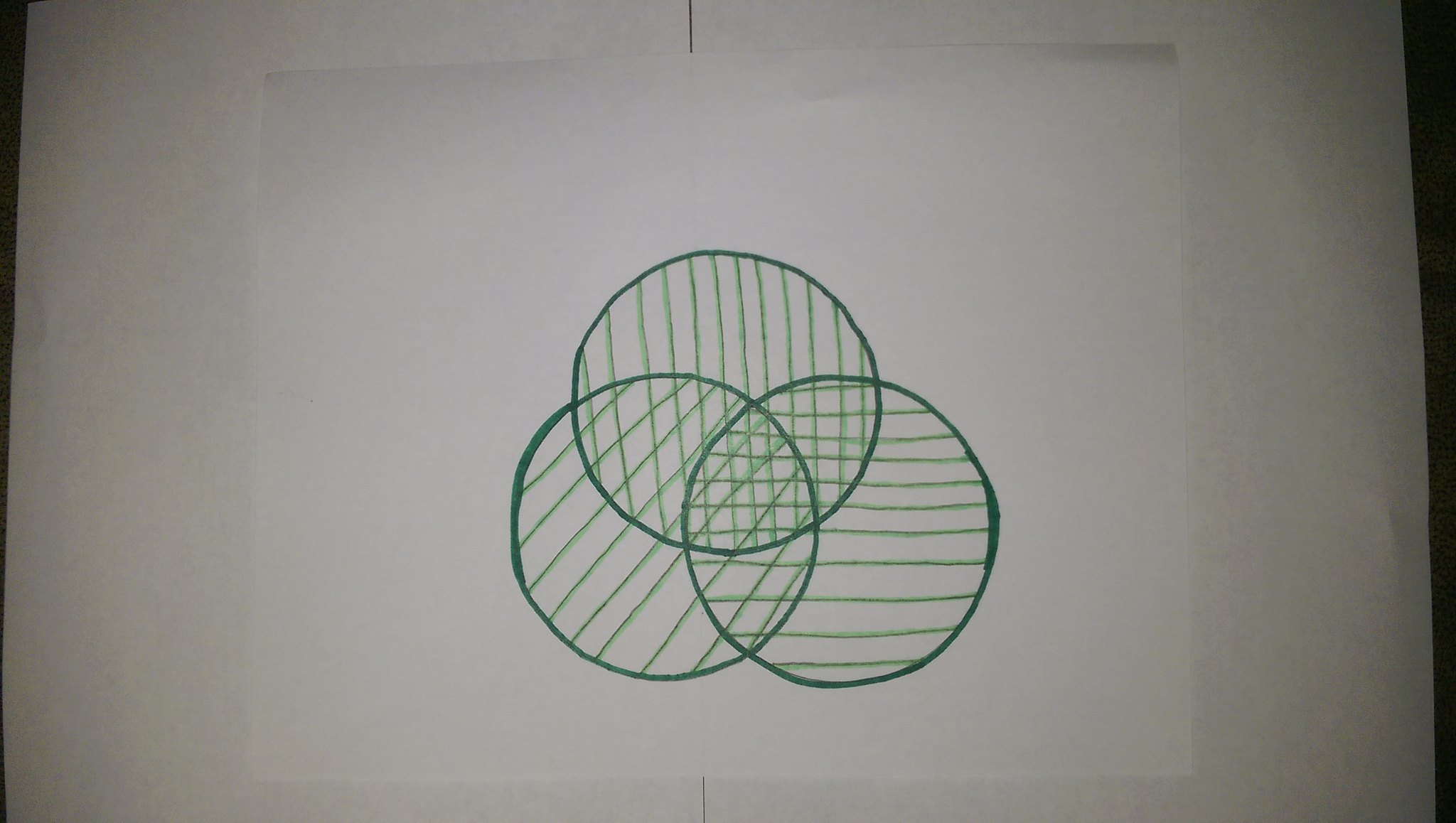This image showcases an artistic drawing on a standard white piece of printing paper, resting on an equally white desktop. The drawing consists of three overlapping circles, meticulously drawn with what appears to be a green ink pen or felt-tip marker. Within each green circle, multiple straight lines span from one side to the other, intersecting and creating a dynamic, checkered pattern. As these circles overlap, the lines within them intertwine, forming increasingly dense and intricate square patterns at the intersections, especially towards the center of the composition. The minimalist drawing, devoid of extraneous artistic tools or embellishments, stands out starkly against the plain white backdrop, emphasizing its geometric precision and simplicity.